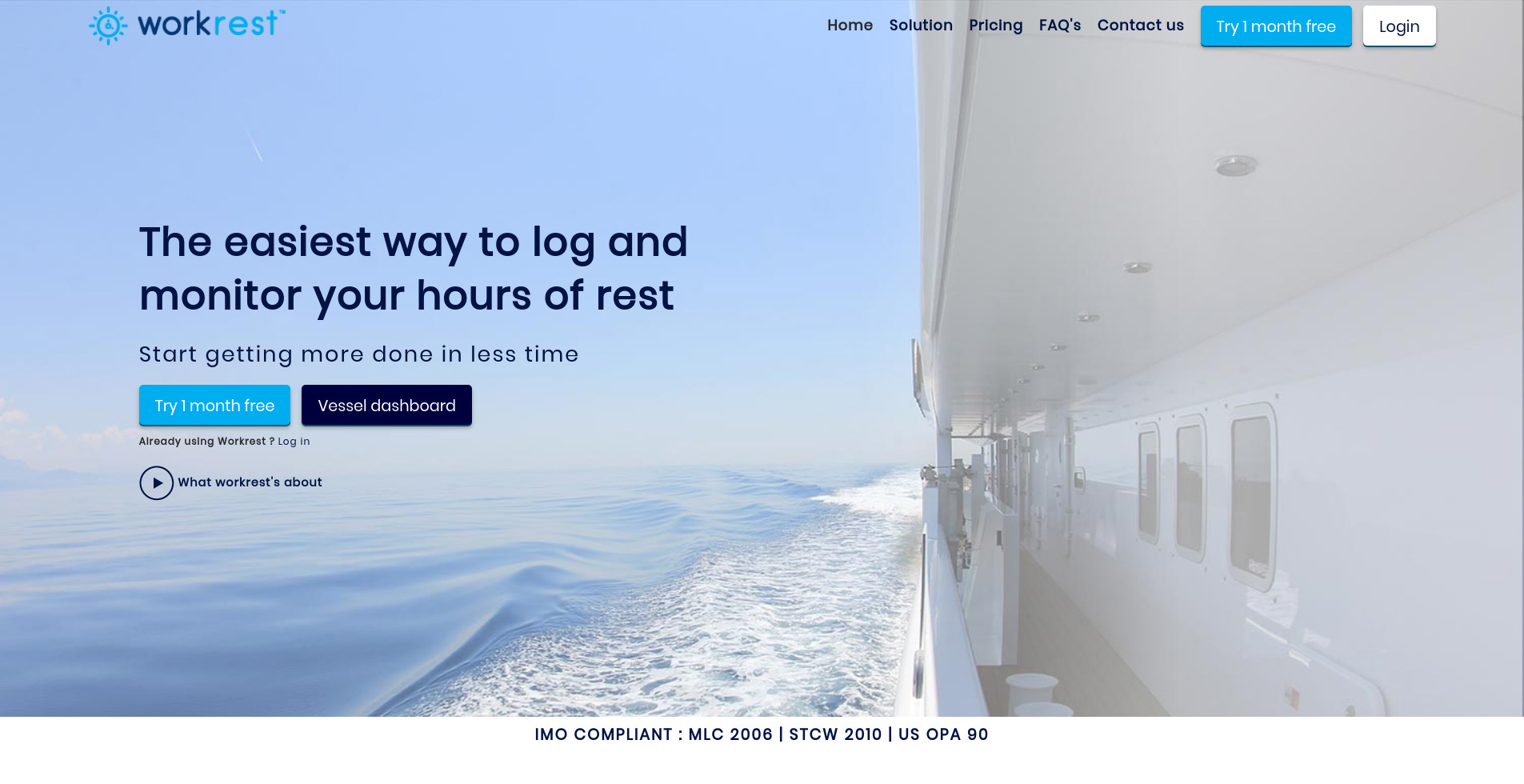The homepage of WorkRest features a striking image that dominates the screen, showcasing the side of a pristine white yacht cutting through the vibrant blue ocean. The sky mirrors the ocean's hue, creating a seamless backdrop, while white waves emanate from the yacht, accentuating its motion.

In the top left corner, the WorkRest emblem, an amalgamation of dark blue and light blue, is prominently displayed. Across the top right, a series of navigation links are aligned in black text: "Home," "Solution," "Pricing," "FAQs," and "Contact Us." 

Beneath these links, a blue rectangular button with bold white text invites users to "Try One Month Free," followed by a contrasting white rectangular button with black text prompting users to "Log In."

Moving down to the middle left, a headline in bold black text declares, "The Easiest Way to Log and Monitor Your Hours of Rest," with a subheadline encouraging efficiency: "Start Getting More Done in Less Time." 

Below this message, another bright blue rectangular button with white text reiterates the offer to "Try One Month Free," followed by a black rectangular button inviting users to access the "Vessel Dashboard." 

Further down, a prompt in black text addresses returning users: "Already Using WorkRest? Log In." Adjacent to this, a black-outlined circle with a directional arrow pointing to the right leads to more information about the platform, captioned "What WorkRest's About?"

Finally, a list of compliance standards is displayed in black text: "IMO Compliant, MLC 2008, STCW 2010, US OPA 90," emphasizing the platform's adherence to international maritime regulations.